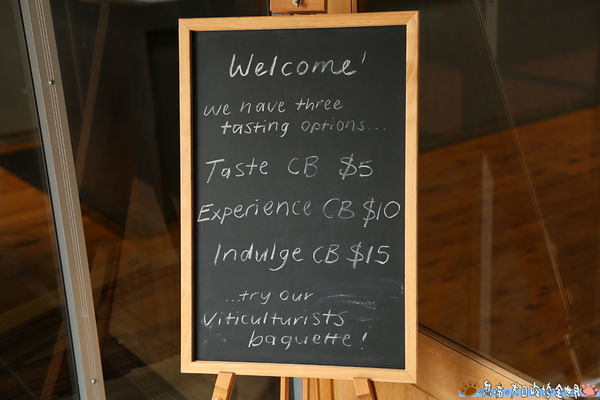This is a detailed photograph of a rectangular, black chalkboard, framed and supported by a wooden tripod stand, positioned at the juncture of two clear windows. The floor beneath and around the chalkboard features beautiful, reddish-brown hardwood, hinting at an older building. The chalkboard, twice as tall as it is wide, delivers a welcoming message in white chalk: "Welcome. We have three tasting options: Taste CB $5, Experience CB $10, Indulge CB $15. Try our Viticulturists' Baguette!" Tiny, indistinguishable pictures decorate the bottom right corner of the board. The overall scene suggests a quaint, possibly vintage pub, restaurant, or bar setting, though the establishment's name isn't visible. The colors captured in the image range from black, white, and gray to silver, brown, pink, and blue, creating a charming and inviting atmosphere.